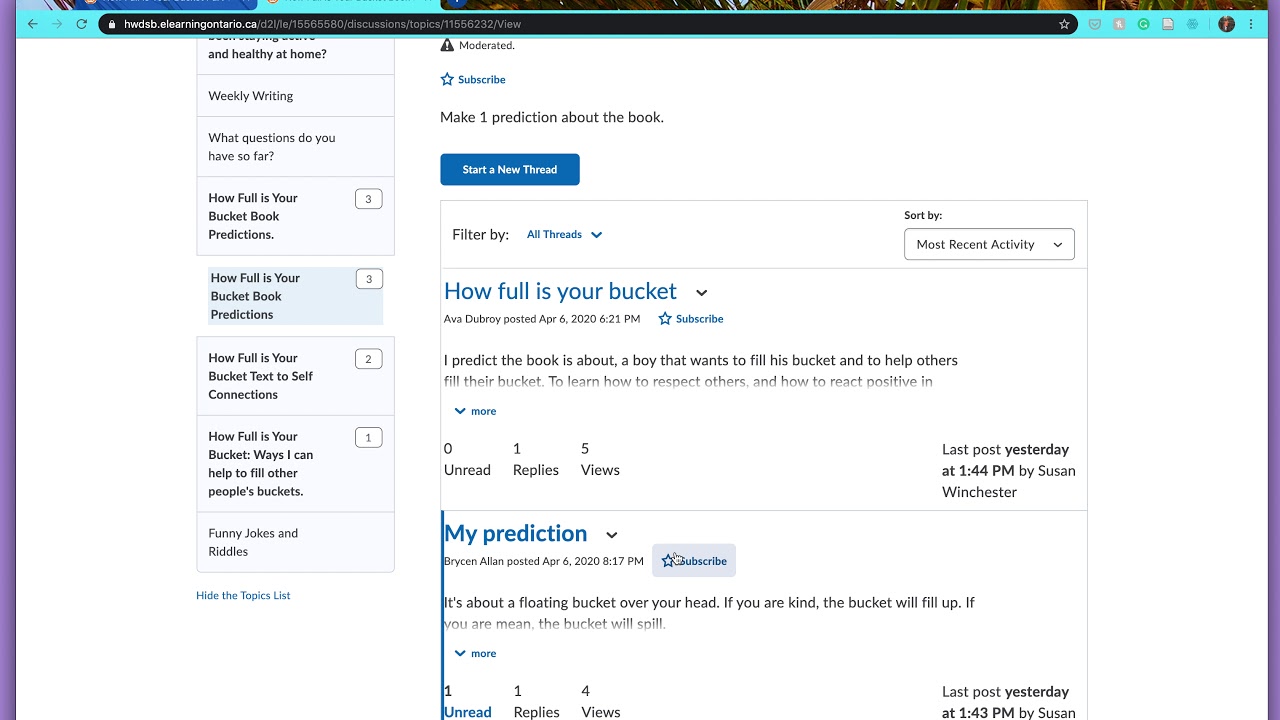This screenshot, though blurry and difficult to read, shows a page from the e-learning website hwdsb.elearningontario.ca, likely operated in Ontario. At the top, there's a search bar with the website's URL. 

On the left side of the screen, a list of options is displayed in a series of rectangles. These options, from top to bottom, are:
1. "Weekly Writing: What questions do you have so far?"
2. "How Full Is Your Bucket: Book Predictions."
3. "How Full Is Your Bucket: Text to Self Connection."
4. "How Full Is Your Bucket: Ways I Can Help to Fill Other People's Buckets."
5. "Funny Jokes and Riddles."

Adjacent to these options, a star icon with blue text reads "Subscribe." Below this, the text prompts users to "Make one prediction about the book." Underneath this prompt, a filter option appears in a rectangle, with black text "Filter by:" followed by the phrase "All the Reds" in blue text alongside a down arrow.

Further down, the screen displays a statement related to the book "How Full Is Your Bucket," suggesting a prediction about the book's content: "Predict the book is about a boy that wants to fill his bucket and help others." Finally, the last rectangle is simply labeled "My Prediction."